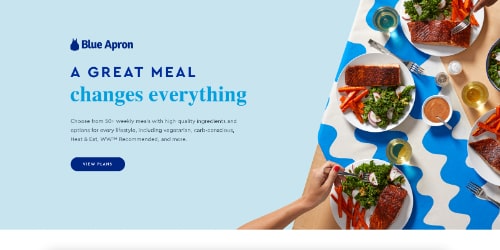The image prominently features a "Blue Apron" advertisement on the left side. The dark blue text reads "Blue Apron" next to the company's logo, a blue apron silhouette. Below, in light blue text, the motto "A great meal changes everything" is displayed. In a very small font beneath the motto, the text reads "Choose from 50+ weekly meals with high-quality ingredients." Further down, a dark blue bubble highlights the words "Meal Plans" in white text.

In the bottom center of the image, a person's arm extends upwards. The individual appears to be a light-skinned woman, recognizable by her red-painted fingernails.

The right side of the image features a light brown wooden table covered with a white tablecloth adorned with blue wave patterns. Set on the table are four plates, each holding a meal consisting of a piece of meat, some carrots, and green vegetables.